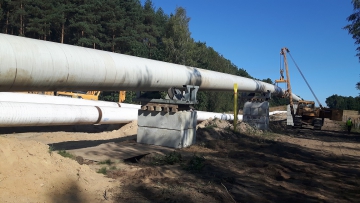This detailed color photograph captures an outdoor daytime construction site. The foreground consists of churned-up, rocky brown dirt with minimal greenery. Two large white pipes extend diagonally from the left edge toward the center of the image, partially supported by big metal and concrete bases. There is a crane or yellow pulley lift machine positioned on the right side, hovering over one of the pipes, indicating active construction work. In the background, a lush green forest dense with tall trees forms a horizon, while the clear blue sky frames the upper right corner of the photo. Notably, there are no people, animals, or buildings visible in the image, nor any legible writing.